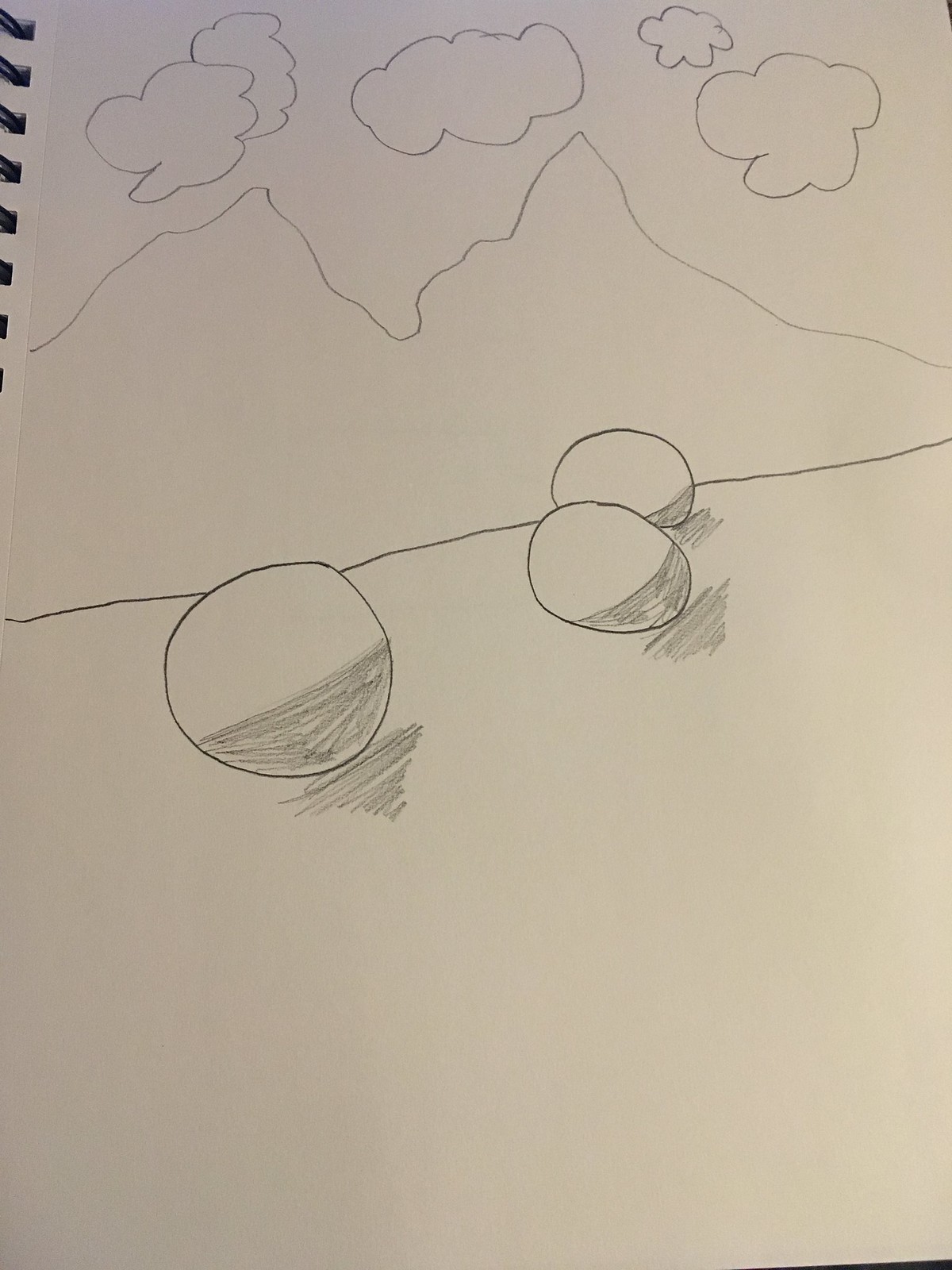This photograph showcases a page from an open sketchbook, with a portion of the black metal spiral binding visible in the upper left corner. The page features a minimalist pencil drawing rendered with simple, yet effective lines. Starting at the top, there are four fluffy, popcorn-shaped clouds spaced evenly across the sky. Below these clouds, two rugged, craggy triangles join together at their bases to form the peaks of mountainous terrain. A horizontal line runs beneath the mountains, demarcating the horizon and the ground. Lower on the page, three circles are neatly drawn, each casting a shadow illustrated by cross-hatching. The lower halves of these circles are shaded in with pencil, adding depth and dimension. The drawing, though basic, conveys a serene landscape with its uncomplicated strokes and straightforward composition.